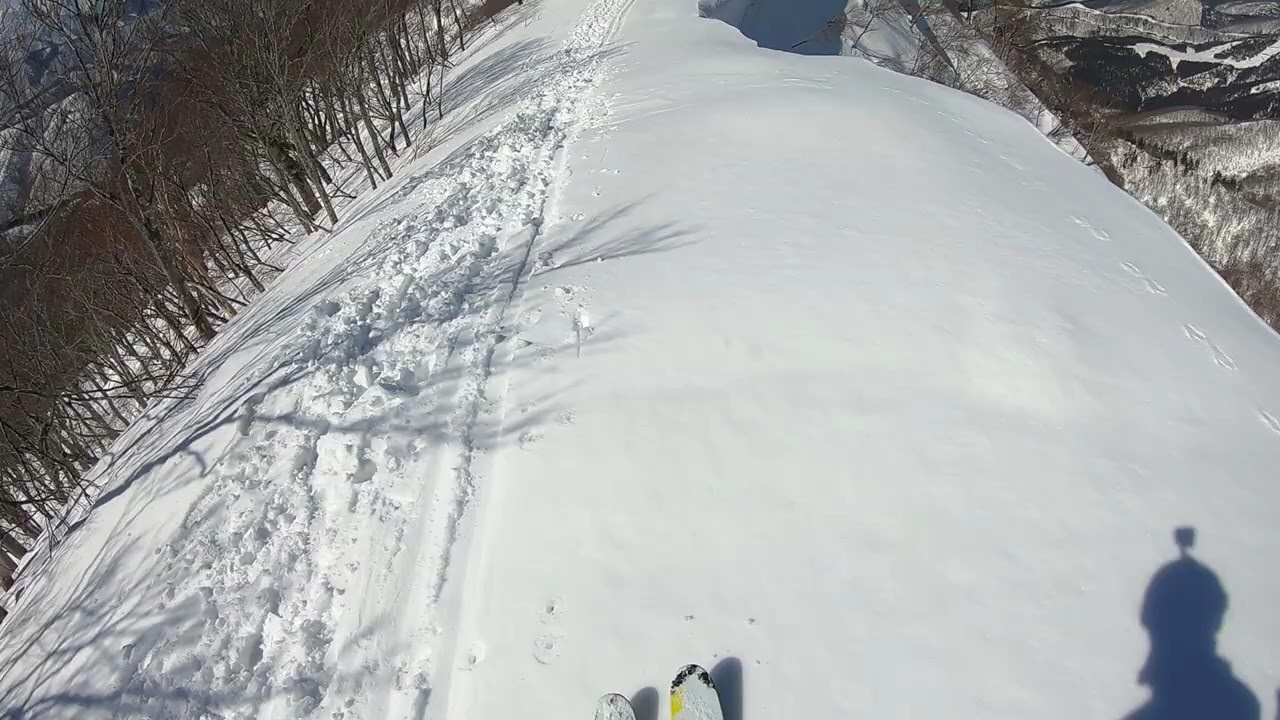The image captures an expansive view from a skier's perspective, taken with a helmet cam during a bright winter day at a ski resort. The skier stands at the top of a very tall and steep snowy slope. The vivid yellow and black tips of the skier’s skis are visible at the bottom center of the frame, slightly dusted with snow. The snow ahead is pristine and white, with a clear section to the right and ski tracks cutting through it to the left, indicating that others have skied down this path. On the left, brown, bare trees with empty branches grow from the side of the slope, angled slightly due to the steep incline. Farther in the distance, more trees and rolling snowy hills can be seen, marking different elevations in the landscape. The sun shines brightly, reflecting off the snow, while behind the skier, the long shadow of the person and their helmet cam stretches into the bottom right corner of the image, emphasizing the height and clarity of the day.